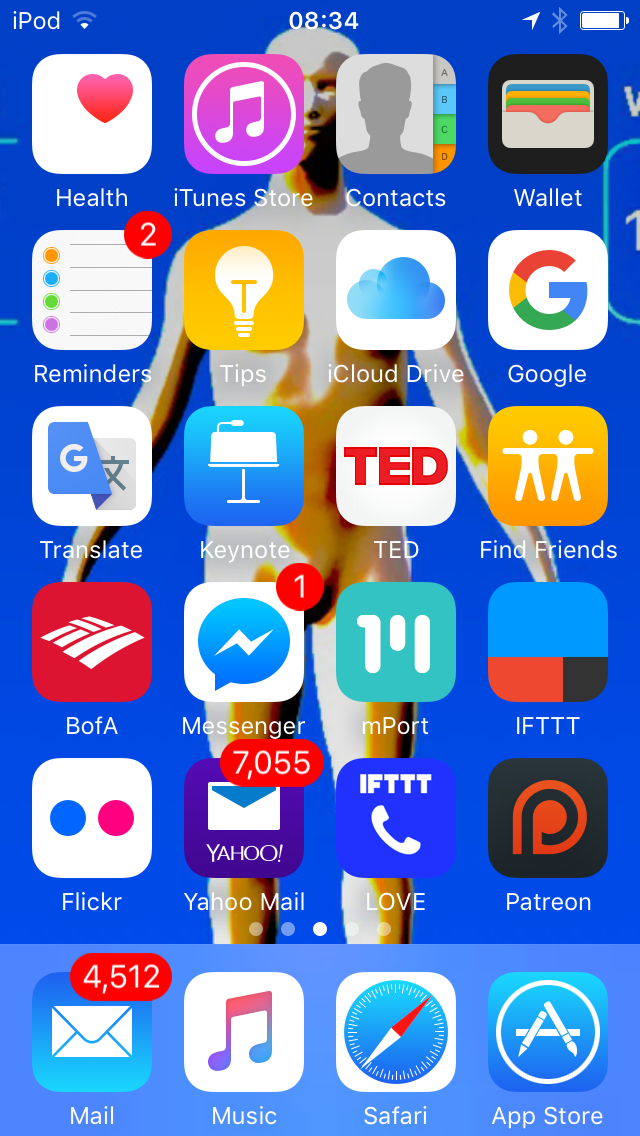This screenshot captures a cell phone screen with a vibrant, blue-themed background featuring a 3D human figure positioned centrally. At the very top left, "iPod" is displayed, indicating the device. In the middle of the status bar at the top, the time reads "08:34," and the top right corner features various status icons.

The main screen layout consists of a grid of app icons, organized into 5 rows of 4 squares each, topped with a clearly defined row separated by a thin blue line. Each icon is distinctly colored and labeled with corresponding text beneath it.

The first row of icons includes:
- Health
- iTunes Store
- Contacts
- Wallet

The second row features:
- Reminders
- Tips
- iCloud Drive
- Google

The third row displays:
- Translate
- Keynote
- Ted
- Find Friends

The fourth row contains:
- Bank of America
- Messenger
- Mport
- IFTTT

The fifth row presents:
- Flickr
- Yahoo Mail
- Love
- Patreon

Separated by a solid blue line, the bottom row features another set of four icons labeled:
- Mail
- Music
- Safari
- App Store